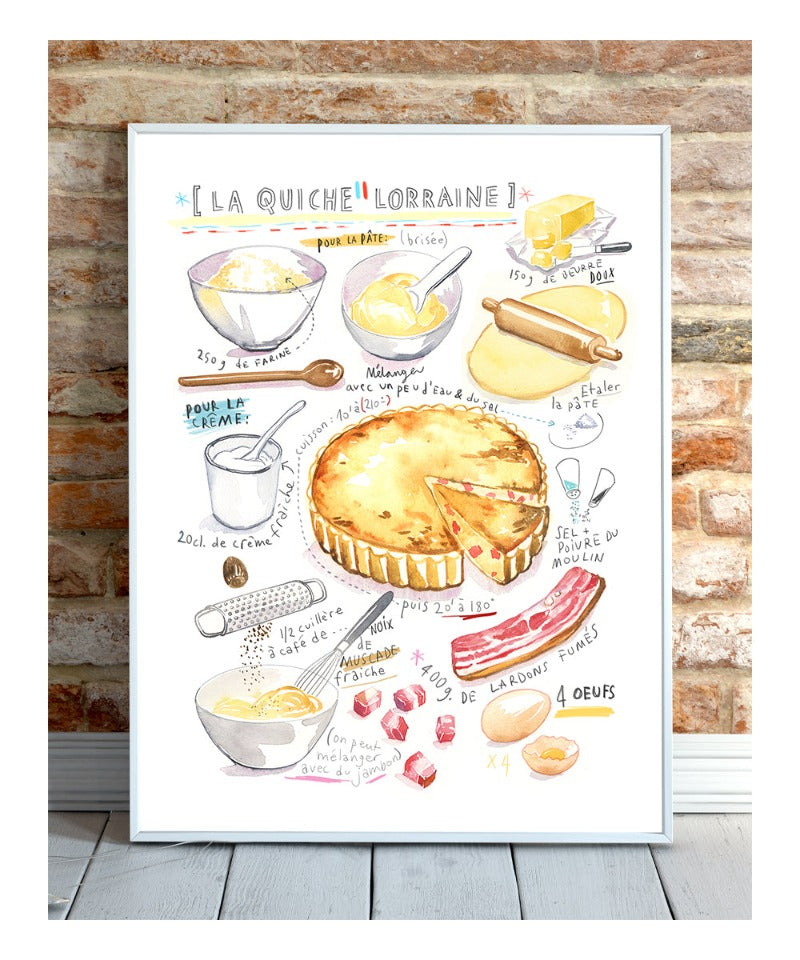The image showcases a meticulously detailed drawing of various food items, set against a crisp white background. At the top, two bowls are prominently featured, one filled and one empty. To the top right, a small collection of baking essentials – a slab of butter, a rolling pin, and some dough – are carefully illustrated. Centrally positioned are a wooden spoon and a cup brimming with cream, accompanied by a beautifully rendered pie and classic salt and pepper shakers. The bottom section reveals a busy assortment of culinary tools and ingredients: a bowl with a whisk poised in motion, a robust grater, a substantial chunk of meat paired with diced meat cubes, and an egg shown both whole and halved. Surrounding each item are words inscribed in a non-English language, adding an air of international flair to the illustration. The background brick wall, awash in shades of light red, orange, with a single starkly dark brick on the right, provides a rustic canvas that contrasts with the white molding at its base. The gray wooden floorboards beneath complete the setting, grounding the vibrant composition in a homely kitchen environment.